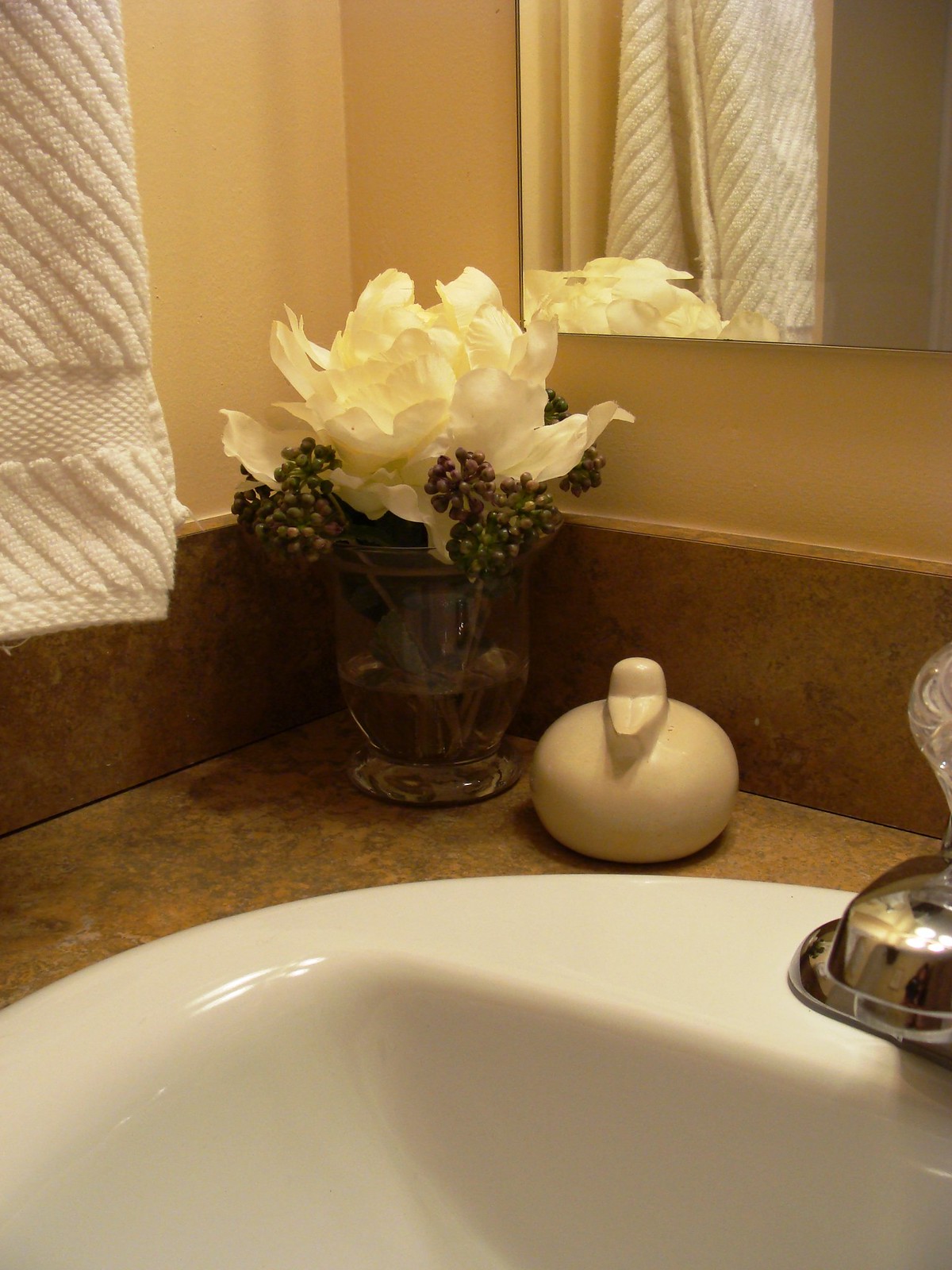In the corner of a bathroom vanity, above a white sink with a curved rim and flat back, a serene scene unfolds. The walls are painted a soothing brownish cream color, complementing the mottled brown countertop that extends upward as a backsplash. A white towel hangs elegantly, though its rack remains unseen.

A short yet wide glass vase, filled with water, sits on the countertop, showcasing a large white flower bloom accompanied by clusters of red berries or perhaps purple flower buds, adding a touch of nature. Next to the vase stands a ceramic duck figurine, evocative of its form but not overly realistic, adding a whimsical charm to the setting.

A large, frameless mirror is mounted on the wall, situated so that it allows glimpses of the brownish cream walls on either side, enhancing the room's sense of space without dominating it. The water faucet is silver and features a clear plastic knob on the hot water side, providing a glimpse into a simpler, functional design.

Though the camera's view is limited, this corner of the bathroom offers a blend of practicality and aesthetic appeal.